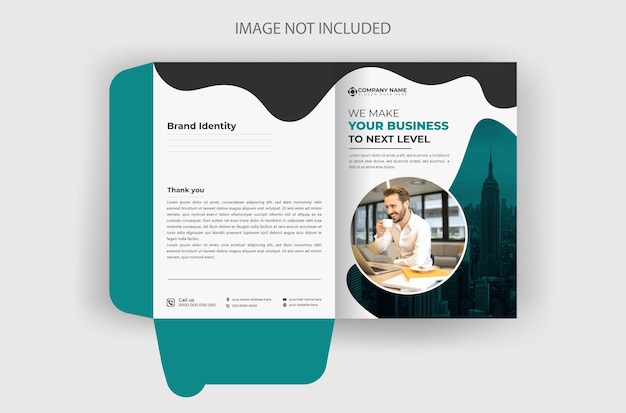The image depicts a detailed promotional pamphlet template with a gray background. On the left page, there is a turquoise border along the left and bottom edges, while the top edge has a black border that forms a series of hills. At the top of this page, "Brand Identity" is prominently displayed in bold letters, followed by four blank lines. Below this section is a thank-you note, additional smaller text, and a delineation with a symbol indicating "Call Us" along with a phone number and other small print. 

On the right page, set against a white background, "Company Name" is presented at the top. Below it, a prominent headline reads, "We make your business to the next level," with "your business" in turquoise and the rest in gray and black. A line underlines "to the next level," followed by smaller text. To the right, there is an image of a bearded man in a white button-down shirt, holding a cup of coffee and facing a laptop. This image is adjacent to a dark, blue-encased picture of a skyscraper, possibly the Empire State Building.

This pamphlet layout, reminiscent of a website or a mailer, features contrasting colors—green, white, and black—throughout its design. The left page's elements fold onto the right, with trapezoidal flaps suggesting the possibility of folding the entire pamphlet into a compact, mailed item.